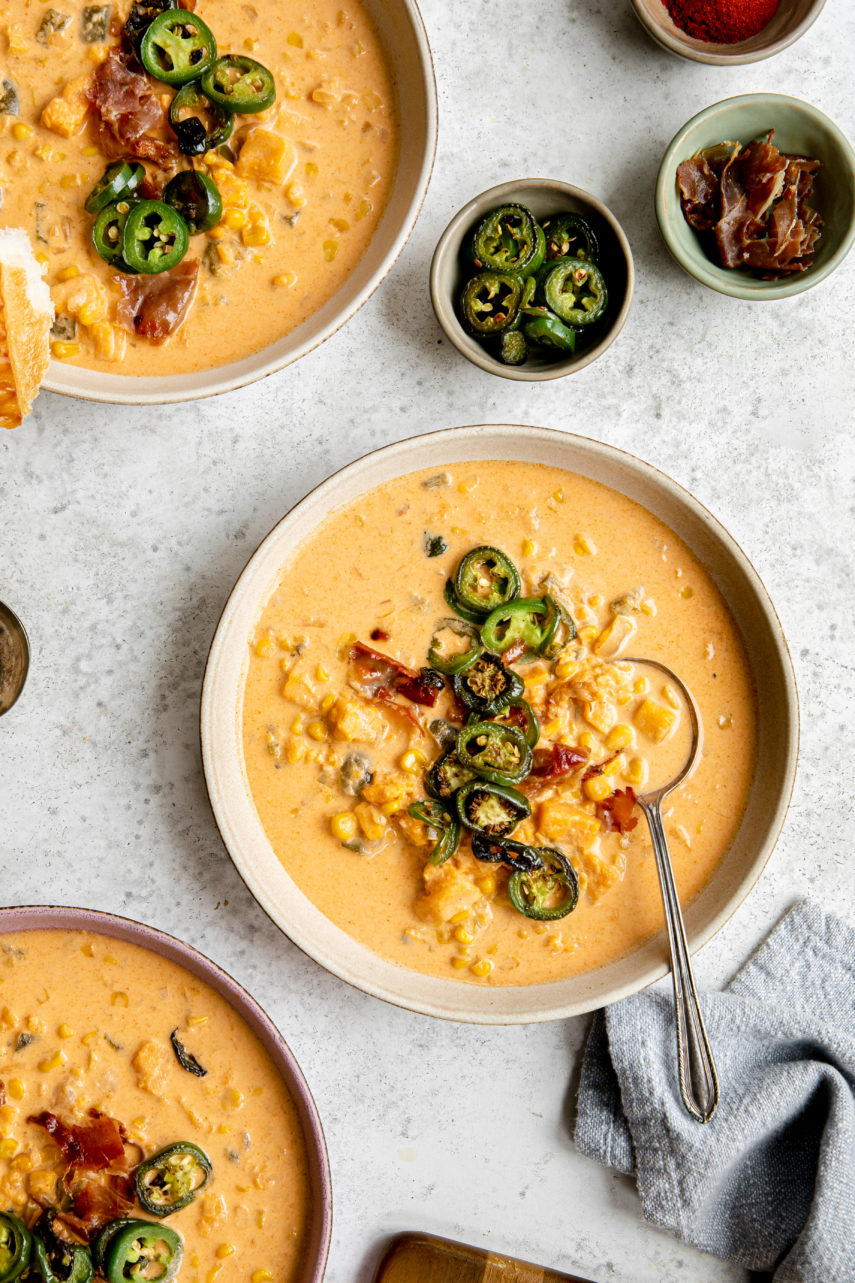This overhead photograph showcases a culinary setup featuring three bowls of the same type of cheddar soup on a speckle-patterned white table. The hearty orange soup, made up of corn, green jalapenos, and bacon bits, fills each bowl uniformly. A silver spoon rests in the center bowl, partially draped over a small gray napkin. Adjacent to the bowls of soup, smaller dishes contain individual ingredients such as sliced green jalapenos and crispy bacon strips, ready for additional garnishing. A glimpse of a wooden cutting board is visible at the bottom corner, adding a rustic touch to the sophisticated setup that might be straight out of a recipe book.